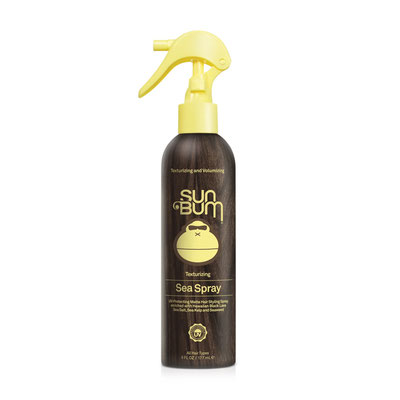In this product photograph, a single object, a spray bottle of Sun Bum Texturizing Sea Spray, is prominently displayed against a pristine white background, creating the illusion of it floating in a white void. The bottle, centrally positioned, is oval-shaped and crafted from brown plastic designed to mimic wood grain, standing straight up in perfect condition, suggesting it is unused. The spray cap, a bright banana-yellow color, features a little trigger and a tiny nozzle, oriented to the left. The front of the bottle showcases multiple lines of yellow text, reading "Sun Bum Texturizing Sea Spray" alongside a distinctive monkey face logo wearing what appears to be sunglasses. This meticulously styled product image emphasizes the bottle's sleek design and brand details, making it suitable for retail listings on websites like Walmart or Amazon.